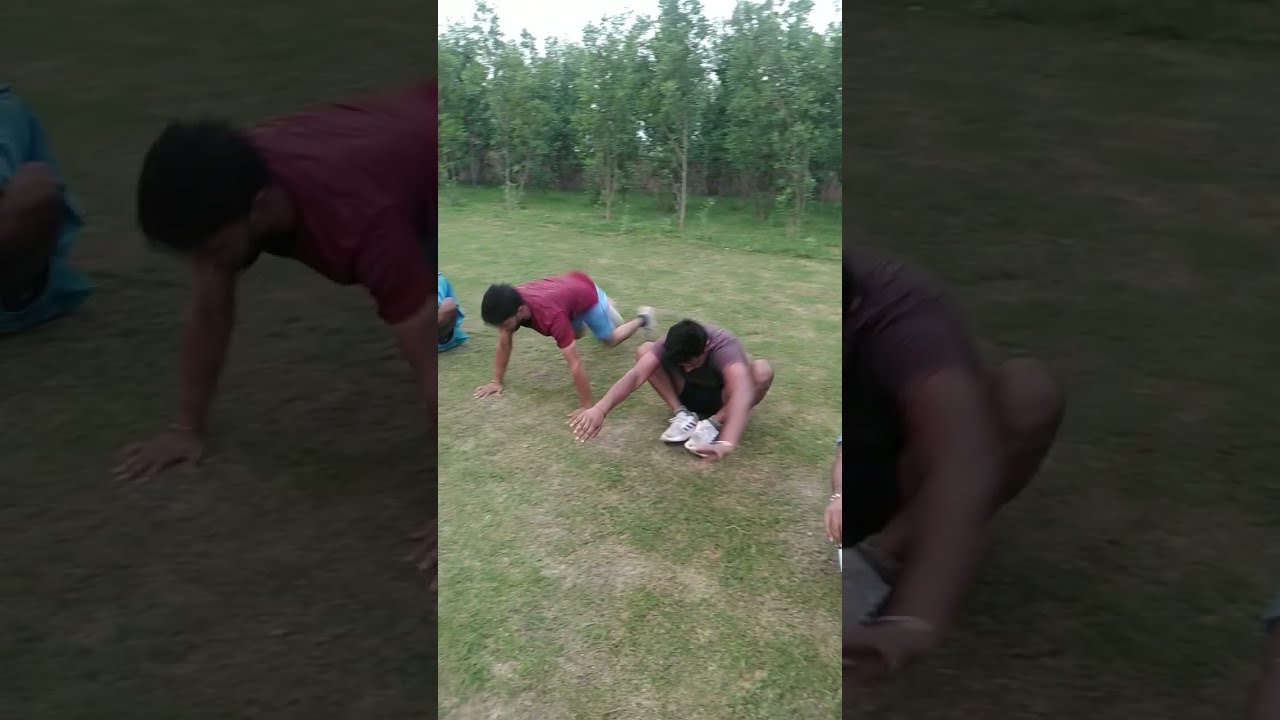The image appears to be a still from a phone video captured in portrait orientation, showcasing three Indian men engaged in exercise routines on a dry, grassy lawn surrounded by tall green trees under a clear blue sky. The leftmost individual is almost out of the frame, with only part of his shirt and knee visible. The central figure, a young man with dark brunette hair and a beard, is bent over with extended arms, assumedly about to perform a push-up. He sports a red t-shirt and blue shorts. The rightmost participant, identified by his dark hair and wearing a brown t-shirt with black shorts and white shoes, sits on the ground performing butterfly squats with his knees spread apart and feet together. Despite the fragmented view, the scene focuses centrally on these individuals, emphasizing their exercise activities amidst the natural, tree-filled setting.